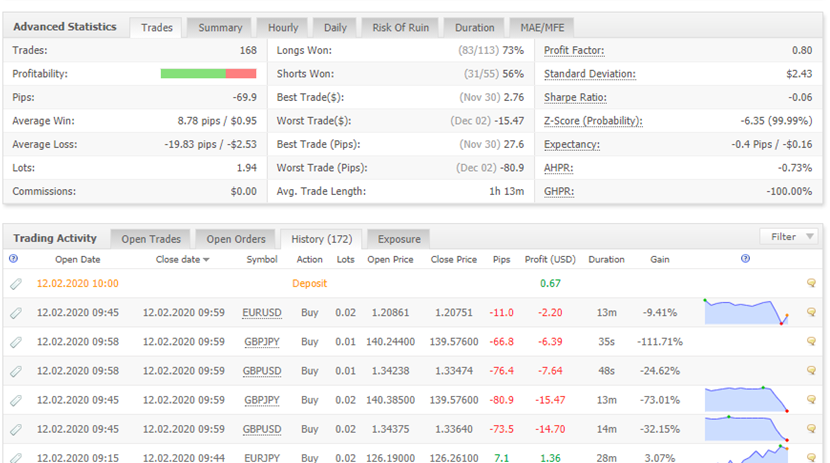**Caption:**

The screenshot showcases a detailed view of advanced statistics and trading activity within a trading platform. The interface is set against a white background with dominant gray elements. At the top, a gray bar displays various clickable menu options, including "Trade," "Summary," "Hourly," "Daily," "Risk of Ruin," "Duration," and "MAE/MFE." The "Trades" tab is currently selected.

Beneath the menu bar, the trades window is divided into three distinct segments filled with numerous entries and statistics:

1. **Trades Summary:**
   - **Trades:** 168
   - **Profitability Bar:** A bar is half-filled with green, indicating the profitability rate.
   - **Pips:** -69.9 (negative)
   - **Average Win:** 8.78 pips or $0.95
   - **Average Loss:** -19.83 pips or -$2.53
   - **Lots Traded:** 194
   - **Commission:** $0

2. **Longs/Shorts Performance:**
   - **Longs:** 1 trade, 73% success rate
   - **Shorts:** 1 trade, 56% success rate
   - **Best Trade:** 2.67 (presumably in pips or currency unit)

Each segment provides a clear and concise overview of different aspects of trading activity and performance, making it an essential analytical tool for traders.